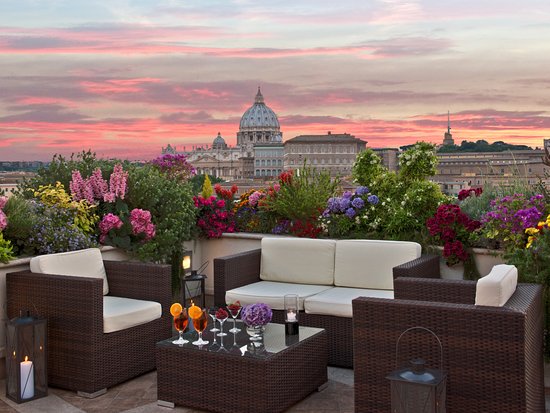This image captures a stunning rooftop balcony at sunset, providing a breathtaking panoramic view of a cityscape dominated by historical 18th-century buildings, including a prominent domed capitol building. The sky is a beautiful gradient of blue, pink, and purple hues, with an orange glow enhancing the clouds as the sun sets.

The outdoor space is elegantly furnished with a brown rattan seating arrangement, featuring a love seat and two individual club chairs, all adorned with white cushions. In the center, a matching coffee table holds an assortment of beverages, including two iced teas garnished with orange slices and several martini glasses filled with cocktails.

Surrounding the seating area, vibrant planters brim with a diverse array of blooming flowers. Rich in colors, the flowers range from yellow daisies, red roses, and pink blooms to purple lilacs, light blue blossoms, and lavender flowers, adding bursts of color that contrast beautifully with the furnishing and the surrounding cityscape.

Candles are thoughtfully placed around the seating area, further enhancing the ambiance, making this rooftop balcony an exquisite blend of urban sophistication and natural beauty.